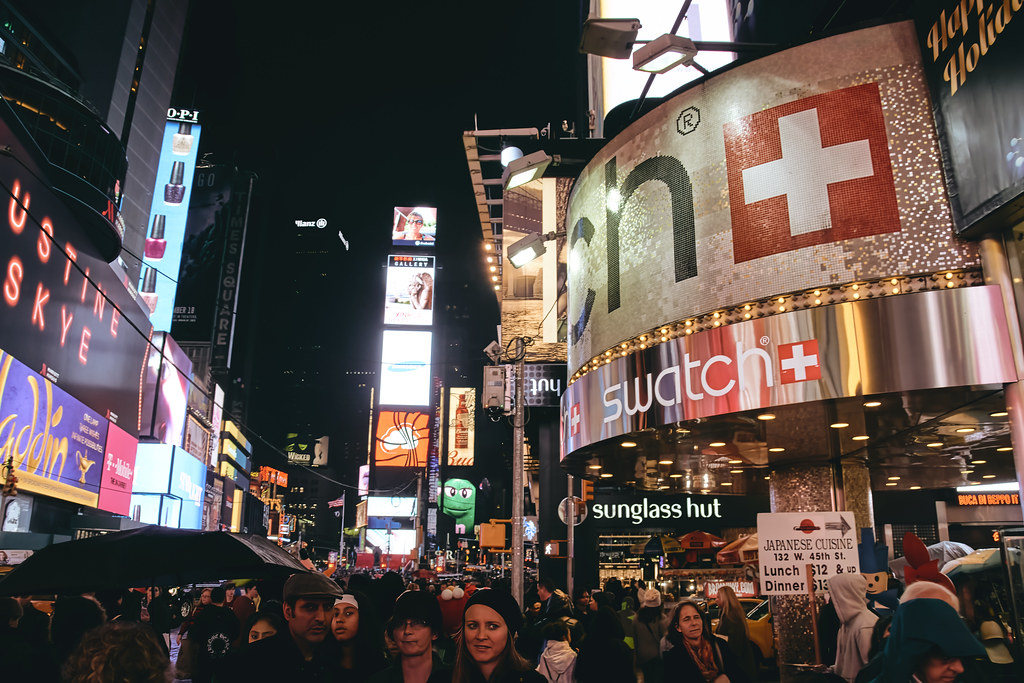This photograph captures a bustling nighttime scene in Times Square, New York City. The sky is a deep black, contrasting with the vivid, illuminated advertisements that line the square. Centered in the image is a tall building, surrounded by a plethora of brightly lit signs and billboards. On the left side, posters for "Aladdin" and a movie poster for "Sky" are visible, while on the right, advertisements for Swatch Watch and Sunglass Hut can be seen, along with a sign for Japanese cuisine. A diverse crowd fills the bottom portion of the image, their heads and shoulders visible under the glow of the advertisements. Notably, one person in the lower left corner holds an umbrella, indicating it is raining. The scene is vibrant, chaotic, and full of life, reflecting the iconic energy of Times Square.